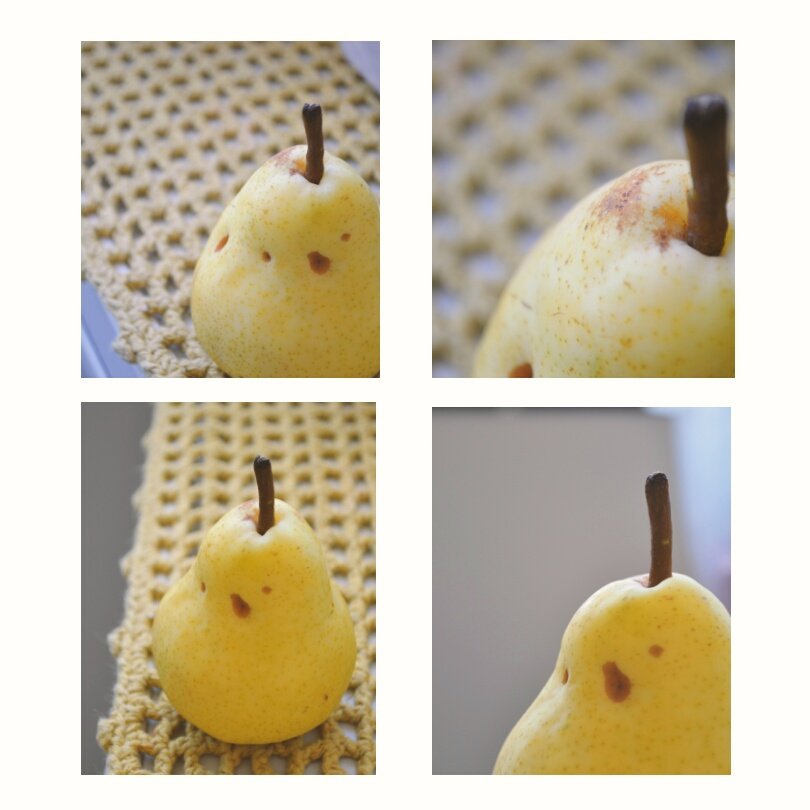This digital collage features a series of four detailed photographs of the same yellow pear, artfully placed against a crocheted cream-colored mat. Each photo is arranged in a square, divided by white borders. In the upper left image, the pear is positioned in the bottom right corner, showcasing its distinctive brown spotting and a small black stem, all set against the textured crocheted background. The top right photo offers an extreme close-up of the pear's top section, where the stem area dominates the frame and the crocheted mat fades into a blurred backdrop. The bottom left photograph presents a more pulled-back view, capturing the entire pear and highlighting three visible brown spots, all resting on the cream-colored mat. Lastly, the bottom right image zooms in again, displaying approximately half of the pear with its brown spots and stem, this time set against a subtly blurred blue background.